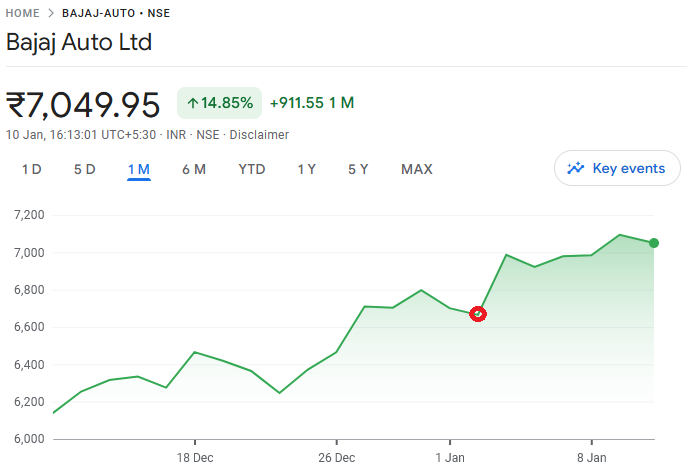The image shows a detailed stock chart from a financial trading page. The background is primarily white, featuring a graph along with various textual elements. In the top left corner, there is a heading: "Home > BAJAJ Auto Limited (NSE)". Directly below, a horizontal line separates this header from the rest of the content.

Beneath this line, there is an unfamiliar currency symbol followed by the value "7049.95". Next to this, a rectangle with an arrow pointing upwards indicates a positive change and reads "14.85%". Adjacent to this is a notation displaying "+911.55" with a small "1M", indicating metrics relevant to the stock’s recent performance.

The lower section of the page contains the chart itself. Above the chart are tabs labeled "1D, 5D, 1M (underlined), 6M, YTD, 1Y, 5Y, Max", offering different timeframes for viewing the stock's performance.

The left vertical axis of the graph shows price levels at intervals: 7200, 7000, 6800, 6600, 6400, 6200, 6000. The bottom horizontal axis provides dates: 18 December, 26 December, 1 January, and 8 January. The stock’s trajectory is depicted with peaks and valleys, starting at just under 6200 and rising to its current value near 7000. A red circle highlights a specific data point slightly above the 6600 mark, shortly after 1 January.

The timestamp "10 January 16:13:01 UTC+5:30" along with "INR - NSE disclaimer" is noted beneath the chart.

This comprehensive visualization encapsulates the stock performance of Bajaj Auto Limited over a selected period, reflecting significant fluctuations and growth trends.